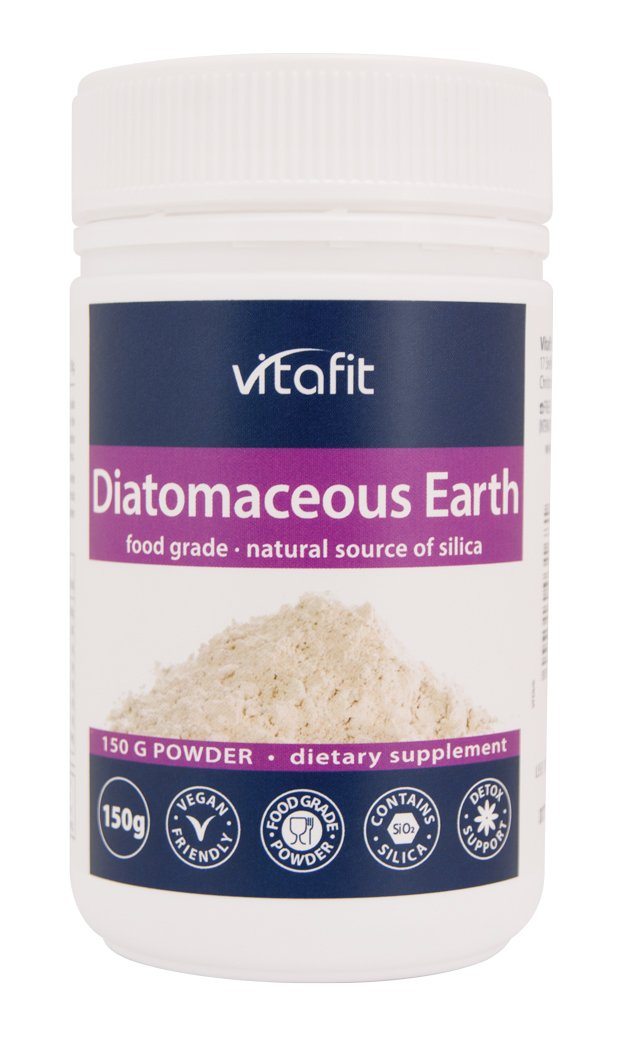The image is a color photograph of a plastic jar containing diatomaceous earth, labeled as a dietary supplement. The jar is white with a striated, screw-on lid and a detailed label on the front. The top of the label features a black band with the brand name "VitaFit" in white letters. Below that, a purple band reads "Diatomaceous Earth" in white lettering. The label further describes the product as "Food Grade, Natural Source of Silica" on a white background, accompanied by an image of off-white powder. A purple band at the bottom states "150G Powder Dietary Supplement." Surrounding this information are several logos indicating "150G," "Vegan Friendly," "Food Grade Powder," "Contains Silica," and "Detox Support." The bottle is set against a white background, emphasizing the product's distinct labeling in shades of blue, purple, and black.